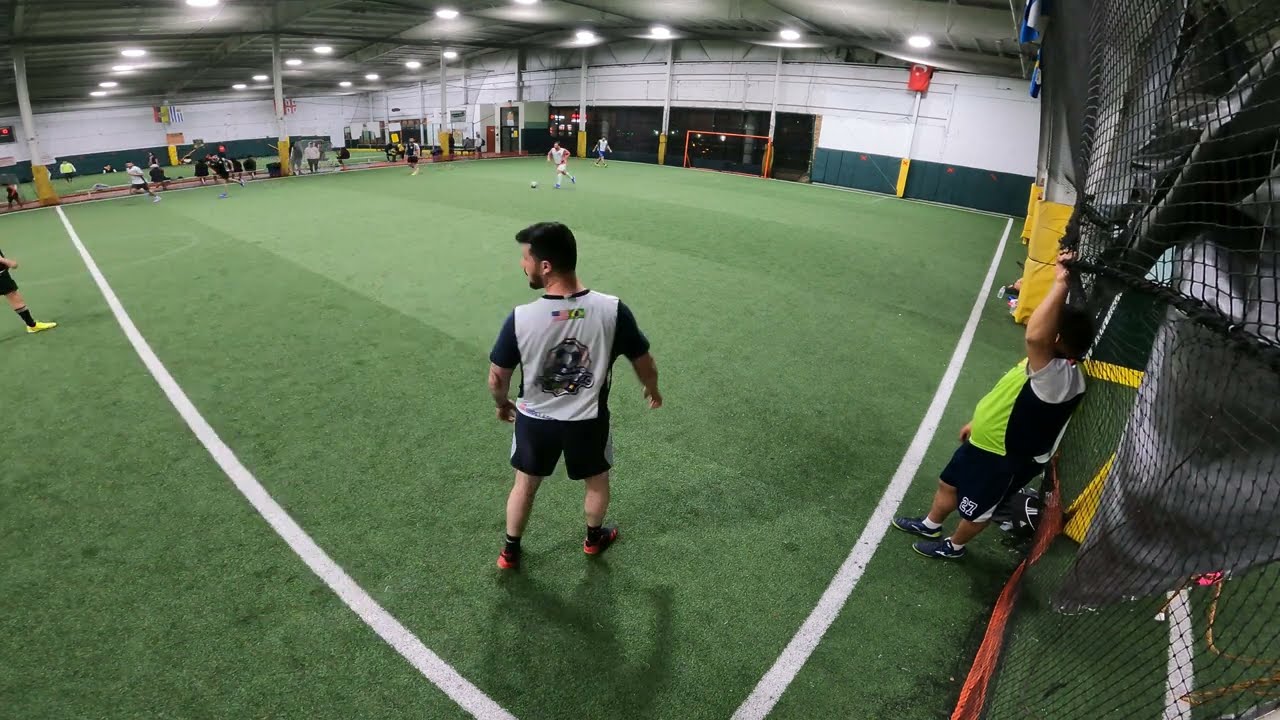This photograph captures an indoor soccer practice or game, likely taken with a fisheye lens that gives it a slight curved perspective. The facility is well-lit by bright fluorescent lights, revealing an expanse of green artificial turf bordered by white lines. The field is enclosed by white walls with exposed metal bars and piping, and blue padding runs around the periphery for safety, complemented by white columns wrapped in yellow padding.

In the center foreground, a young man with dark hair and a beard, wearing a black and white jersey, black shorts, and black and red cleats, looks to his left. He stands near a black mesh netting, and beside him is a man gripping the net. This could be an official, identifiable by some sort of yellow vest.

In the background, a player in a white uniform is seen advancing the ball towards the opposite goal. Scattered across the field are at least three other players—two in black kits and one in white—suggesting active gameplay. On the sidelines, additional individuals in similar colors either watch or prepare to participate, underscoring the dynamic atmosphere of this indoor soccer event.